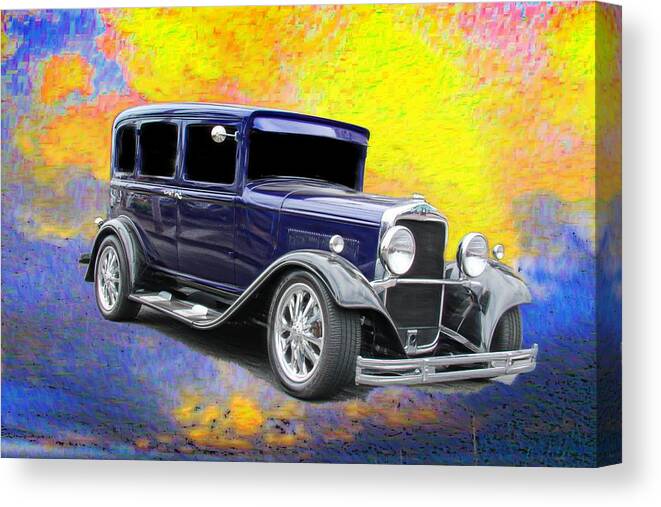This is a horizontally aligned rectangular painting displayed as if for sale, with the edges of its inch-thick canvas visible, casting slight shadows. The background features a dynamic mix of splotchy paint in tie-dyed colors with large yellow areas blended with pinks, reds, blues, and oranges, particularly in the upper left area. The lower part of the painting showcases varying shades of blue with hints of orange, resembling flames. Dominating the center of the canvas is a photorealistic or possibly photographic representation of an old-style car, potentially a Model T from the 1930s. This dark navy blue car is depicted with meticulous detail, featuring shiny chrome bumpers, silver sideboards, rims, and headlights, and black tires. The car appears almost new, standing out vividly against the vibrant, abstract background.